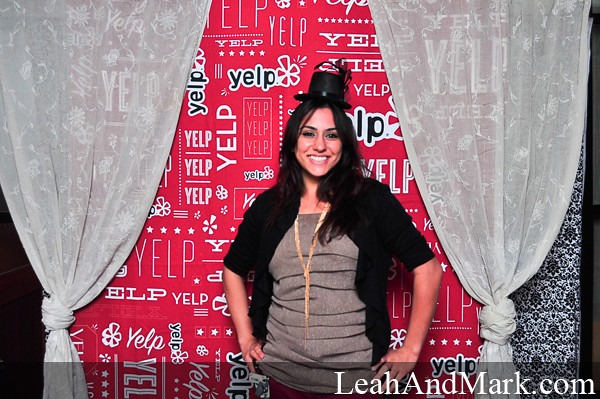In this horizontally aligned rectangular picture, a woman stands facing the camera, smiling broadly and showing her teeth. She wears a black party hat adorned with small flowers, and her long black hair cascades past her shoulders. She is dressed in a black cardigan over a ruffled gray top, accessorized with a long gold chain around her neck. With her hands confidently placed on her hips, she stands in front of a vibrant red wall adorned with various "YELP" text patterns in both black and white, arranged vertically, horizontally, and diagonally in different fonts and cases. On either side of her are white, lacy curtains tied back, revealing glimpses of a black and white patterned wallpaper behind. In the bottom right corner of the image, the text "leahandmark.com" is visible in white. The setting suggests an event or activity sponsored by Yelp.